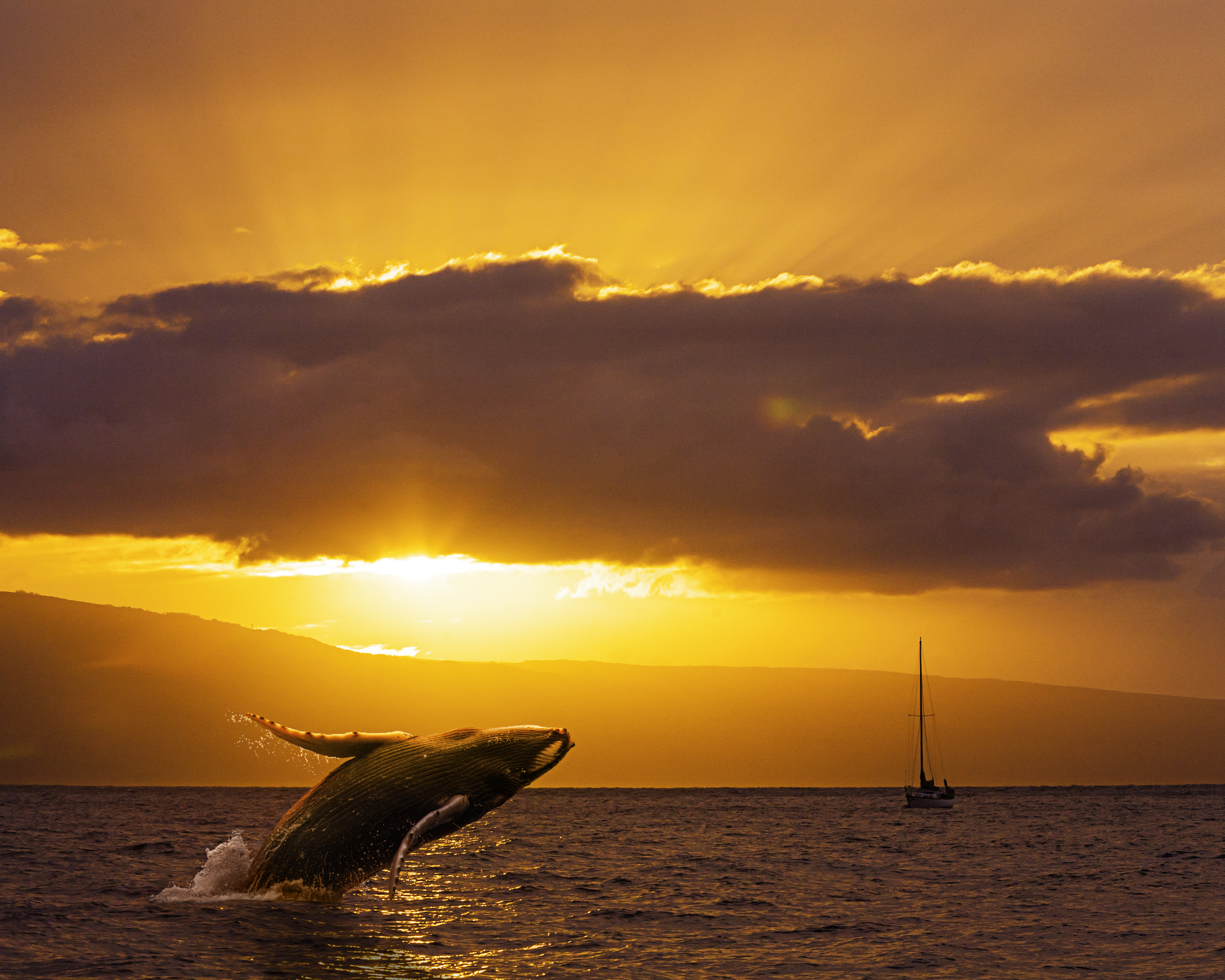In the photograph, a majestic whale is captured mid-breach, seemingly executing an impressive backflip. The whale, substantial in size, soars high above the reasonably still ocean, creating a churning splash at the point where its body leaves the water. This spectacular marine display is set against a dramatic sky painted in deep orange hues, suggesting either sunrise or sunset. Dominating the sky, a massive, dark gray cloud stretches from the left center to the right center, illuminated by the sun positioned behind it. Radiant light rays extend past the edges of the cloud, heightening the atmospheric drama. In the distant right background, a sailboat is visible, its sail not raised, adding a serene nautical element to the scene. A hill or mountain range also presents itself in the far distance, completing this awe-inspiring maritime landscape.